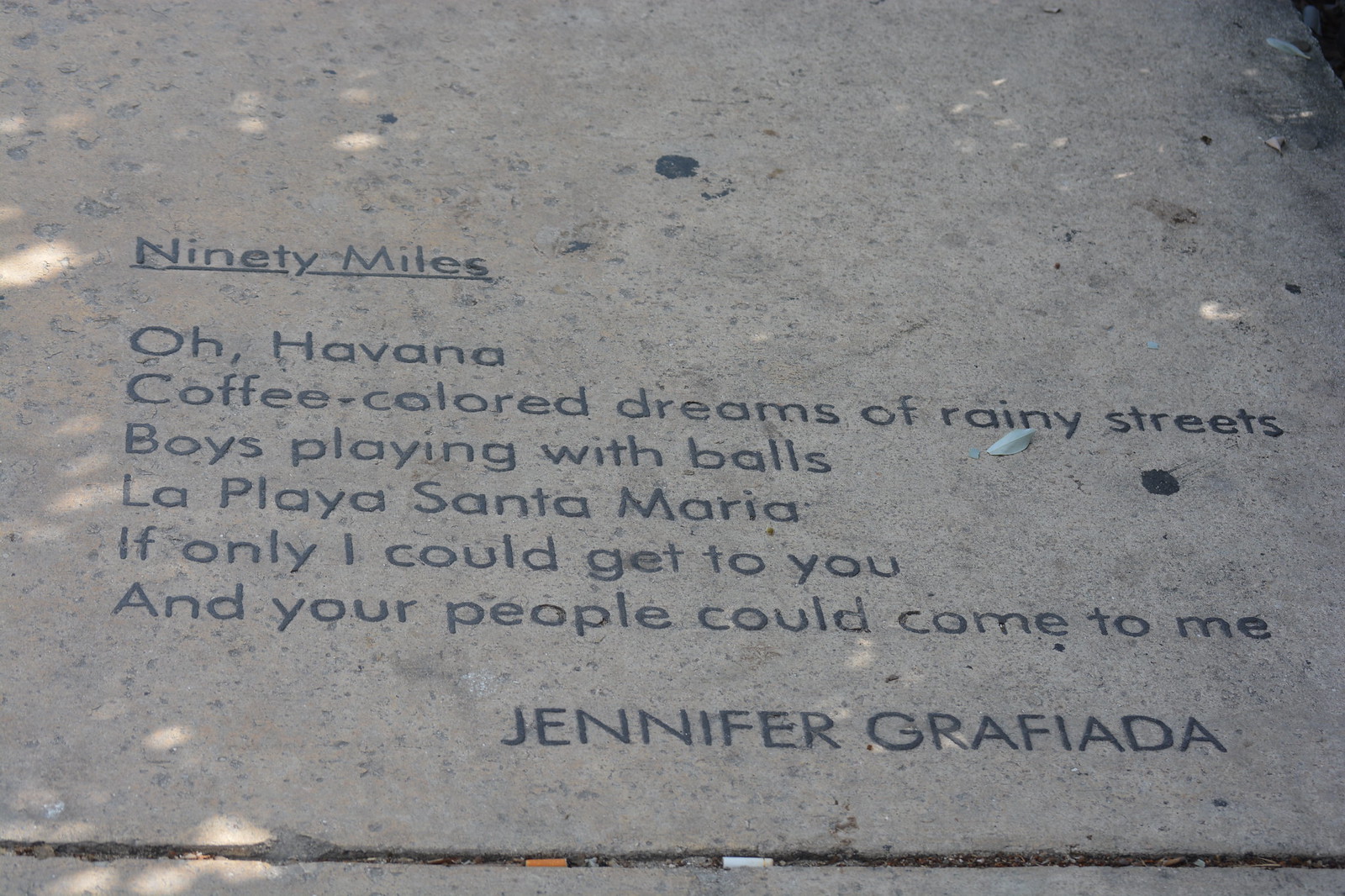On a gritty urban sidewalk, possibly in a park, an engraved monogram reads "90 miles" with an underline, followed by a heartfelt ode to Havana: "Oh, Havana, coffee-colored dreams of rainy streets, boys playing with balls, La Playa Santa Maria, if only I could get to you and your people could come to me." Amidst leaves, cigarette butts, and old gum embedded in the gray concrete, the name Jennifer Grafiotta (G-R-A-F-I-A-D-A) stands out, adding a personal touch to this poignant, poetic tribute. Flecks of sunlight and tree shadows play upon the sidewalk, completing the scene of this evocative urban canvas.